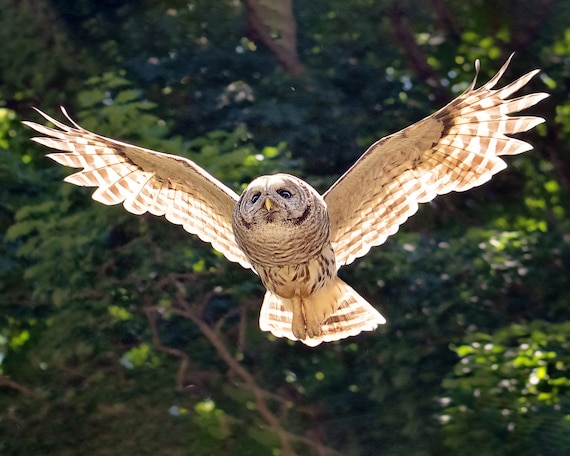In the forefront of this image, an owl with an impressive wingspan is captured mid-flight, its wings spread wide. The owl's feathers display a mix of tan and off-white stripes, while its tail forms a distinct triangular shape. Its expressive eyes, likely dark brown or greenish-blue, appear droopy and possibly focused downwards, possibly at prey. The yellow beak contrasts with its tan-colored body, which features a pattern of dark brown spots scattered across its belly. The owl's wings are remarkable, with the outer edges resembling fingertips, adding to the dynamic feel of the photograph.

Behind the owl, the background showcases a lush forest bathed in daylight. Sunlight reflects off the various shades of green leaves, with some appearing bright and others darker. The forest features an array of thick and thin branches, contributing to the rich tapestry of greenery. The background is slightly blurred, centering the viewer’s focus on the owl's intricate details. The overall scene suggests a vibrant daytime setting, likely captured from a low angle to convey the majesty of the owl in flight, possibly taken by a nature photographer.